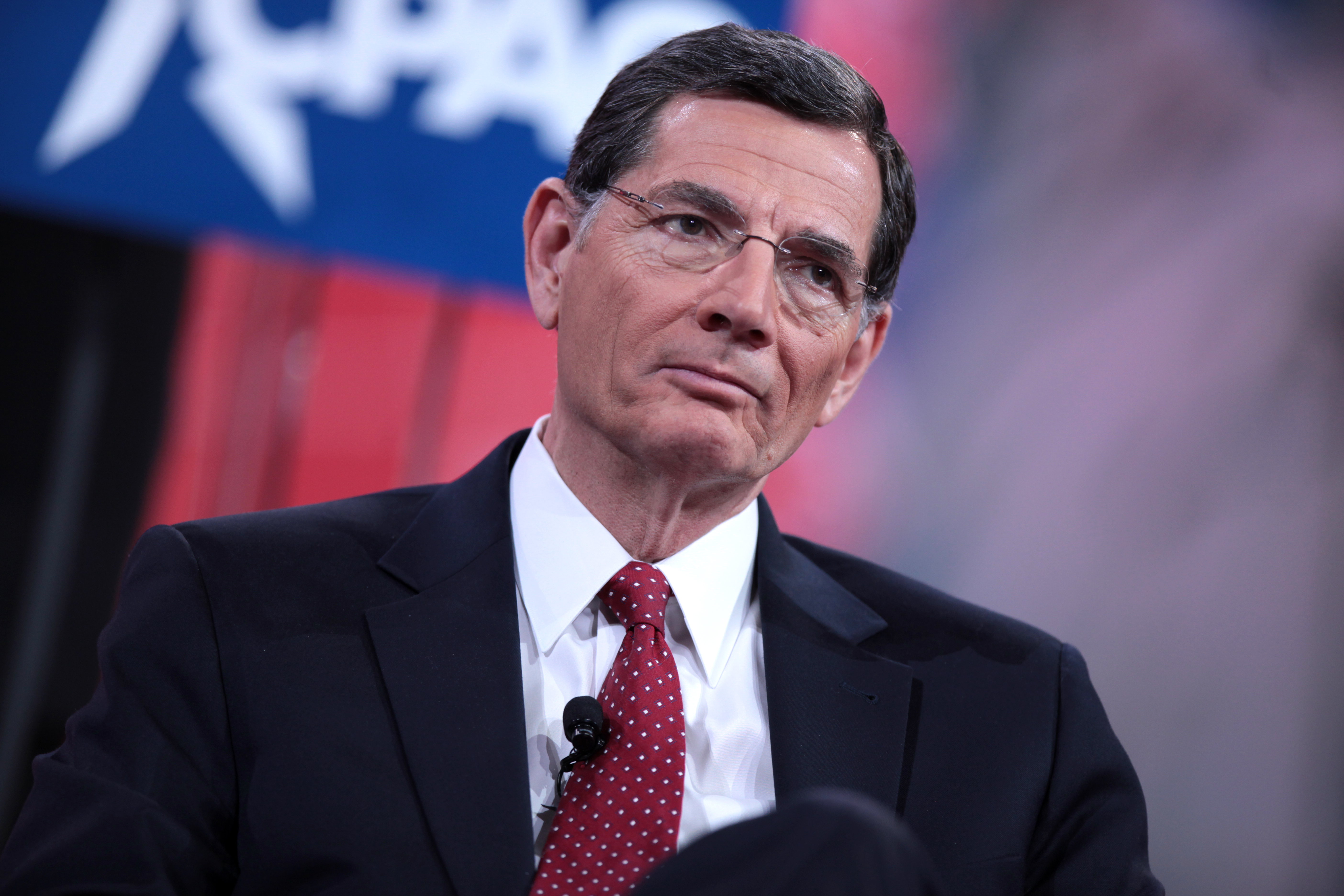In this photograph, we see an elderly Caucasian male, likely in his late 50s to early 60s, who exudes the aura of a politician or someone of significant social status. He is dressed in a classic white button-up dress shirt, a black sports coat, and a distinctive red tie adorned with white polka dots. Completing his professional appearance are rimless glasses and a black clip microphone attached to his tie, suggesting he is speaking at a press conference or similar event. His short brown hair, graying at the sides near his ears, is neatly combed over. The man's expression is serious and somewhat indifferent, as he directs his gaze away from the camera, possibly towards someone asking a question. The background of the image is intentionally blurred, highlighting the subject, but we can discern a blue sign with white capital letters, part of which spells "CPAC," likely indicating he is at a CPAC convention. Additionally, there is a red to black gradient panel and some indistinct purple elements, all set against professional lighting that enhances the photograph's quality.